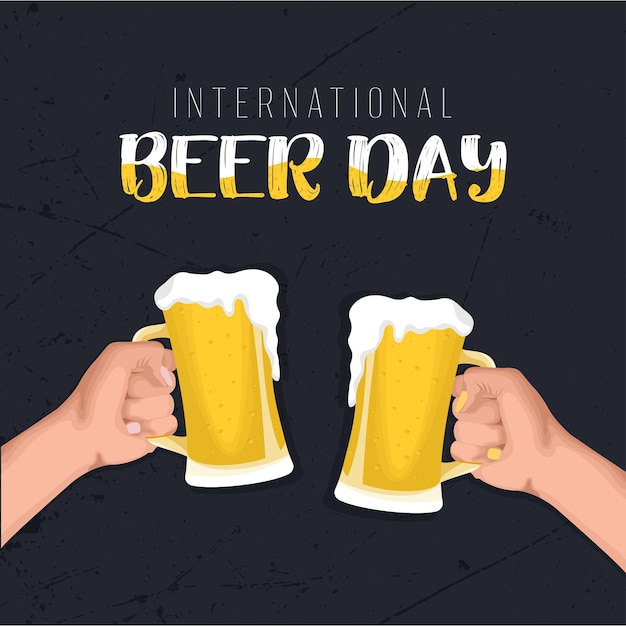The image presents a digitally-created scene with a dark, almost black, splattered background reminiscent of a textured sidewalk. In the foreground, two cartoon-like forearms extend towards each other, each gripping a foamy beer stein. The arm on the right, with medium Caucasian skin tone, has nails painted in yellow, while the arm on the left, also with a medium skin tone, displays light lavender nail polish. The steins, filled with beer, are close but not quite touching, with froth cascading down their sides. At the top of the image, the text "International Beer Day" appears in a chalk-like texture, white at the top and yellow at the bottom, creating a gradient effect that mimics the appearance of beer in a glass.